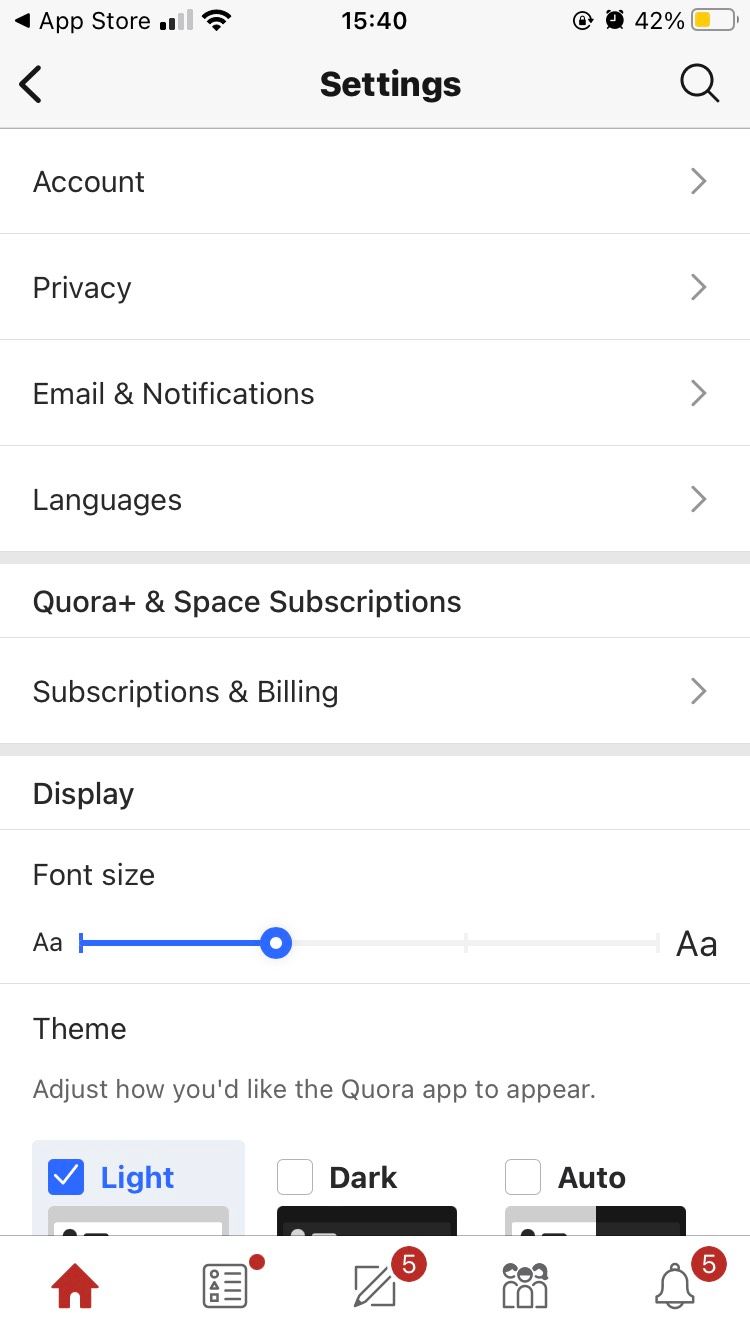This detailed screenshot captures the settings page of an iOS smartphone, distinguished by its clean design and straightforward layout. The interface is predominantly white, with subtle gray shading and bold black text that forms the bulk of the visual elements. Accents of blue appear thoughtfully in checkboxes and scroll bars, adding a splash of color to the monochrome scheme.

Prominently displayed at the top of the screen, the current time reads 15:40 (3:40 PM). The status bar reveals critical information: the device is connected to a cellular network with strong signal strength, has an active Wi-Fi connection, and the battery level stands at 42%. Additionally, the presence of an alarm icon indicates that at least one alarm is set.

The heading "Settings" is boldly highlighted, signifying the active section of the app. Below this, multiple options are neatly listed for user navigation. Key functionalities available on this screen include managing the user's account, privacy settings, email notifications, and language preferences. Other options provide access to Quora and space subscriptions, as well as general subscription and billing information. Furthermore, there's an option to adjust the font size, enhancing accessibility for users.

Overall, the screenshot efficiently conveys the organization and user-friendly design of the iOS settings page, offering a range of customizable options to accommodate the user's needs and preferences.